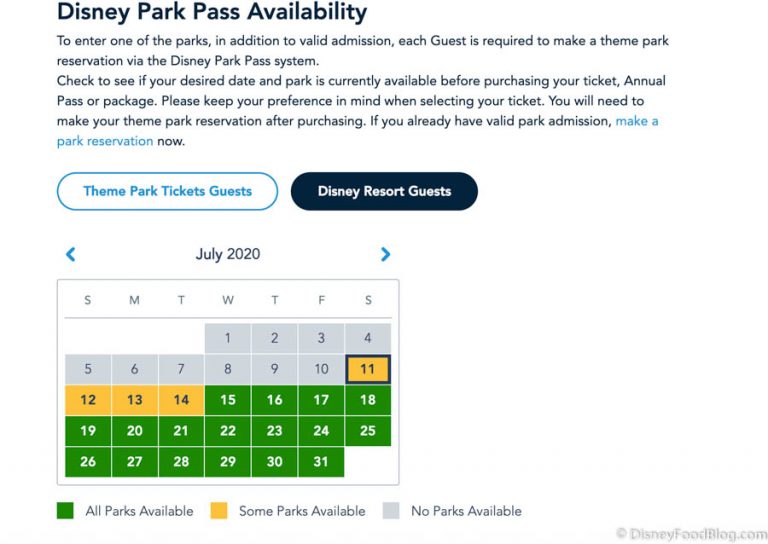The image features a white background with a prominent header in bold black text reading, "Disney Park Pass Availability." Below the header, a paragraph in smaller black text explains, "To enter one of the parks, in addition to valid admission, each guest is required to make a theme park reservation via the Disney Park Pass system." The subsequent paragraph advises guests to "Check to see if your desired date and park is currently available before purchasing your ticket, annual pass, or package. Please keep your preference in mind when selecting your ticket. You will need to make your theme park reservation after purchasing. If you already have valid park admission," followed by a prompt in blue hyperlink text, "Make a Park Reservation Now."

Directly beneath this text, there is a long, white oblong button with a blue border that reads "Theme Park Ticket Guests" in blue lettering. Adjacent to it on the right, a smaller black oblong button displays "Disney Resort Guests" in white text. 

Below these buttons, a calendar is visible, showing the month of July 2020. The calendar's days from the 1st to the 10th are marked in gray, indicating unavailability. Days 11 through 14 are highlighted in yellow, denoting limited availability, while the remaining days are in green, suggesting full availability.